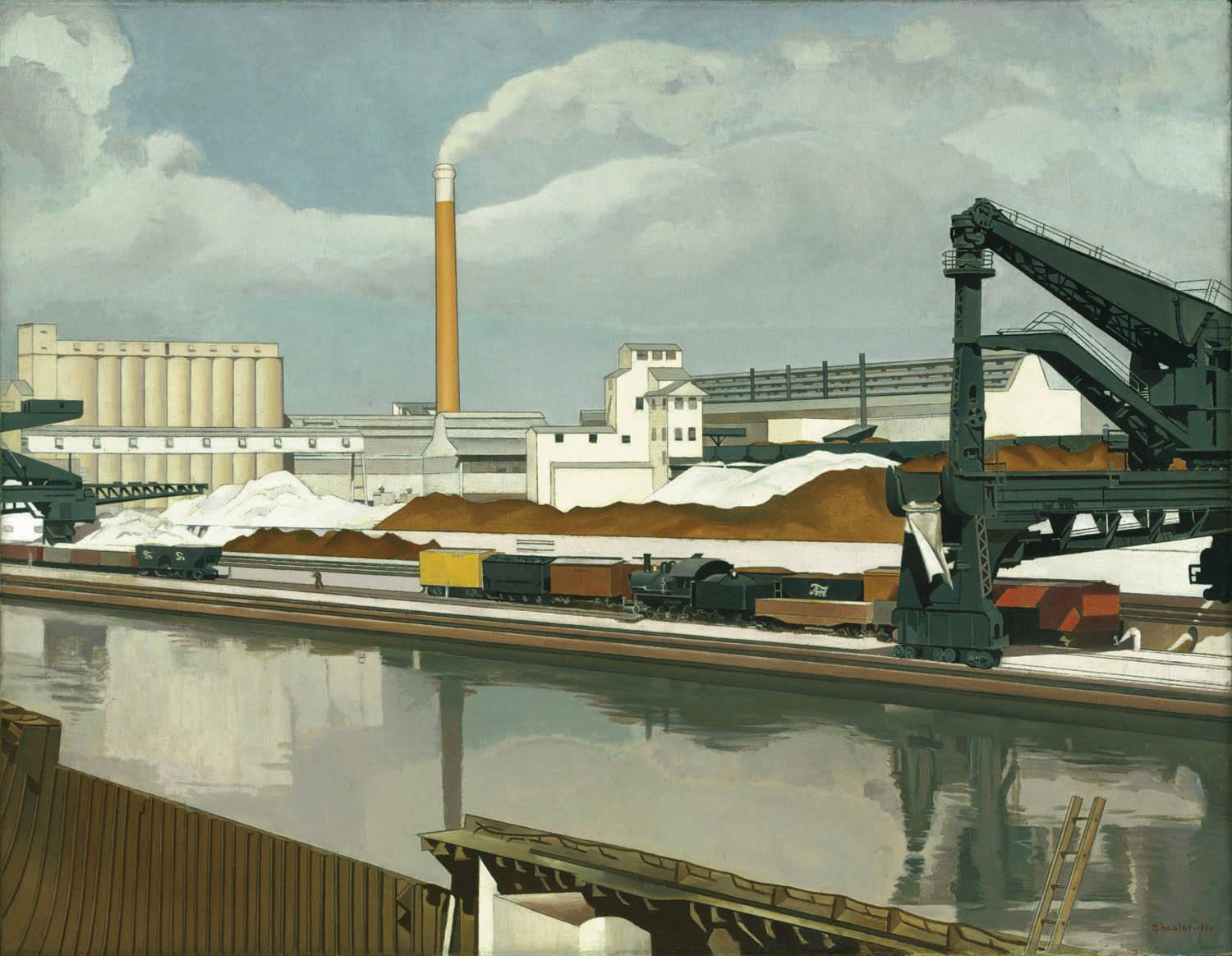The image is a detailed and vibrant drawing depicting a bustling industrial scene, rendered in a smooth, almost three-dimensional cartoon style. The center of the image features a large brown smokestack emitting smoke into a slightly overcast sky filled with blue and giant gray and white clouds. Below, a train with multiple cars - yellow, black, brown, black again, a black car with white writing, rust-colored, and red - runs along tracks parallel to a realistic, light-reflective canal. This canal is lined with hard concrete and industrial machinery, including a dark gray or black crane on the right. The train, possibly a steam engine being loaded, is accompanied by mounds of brown dirt, various containers, and a green crane structure. In the distance, the backdrop is dominated by solid white buildings and hills, with an overall grayish-blue and brown undertone that gives the scene a cohesive industrial atmosphere.